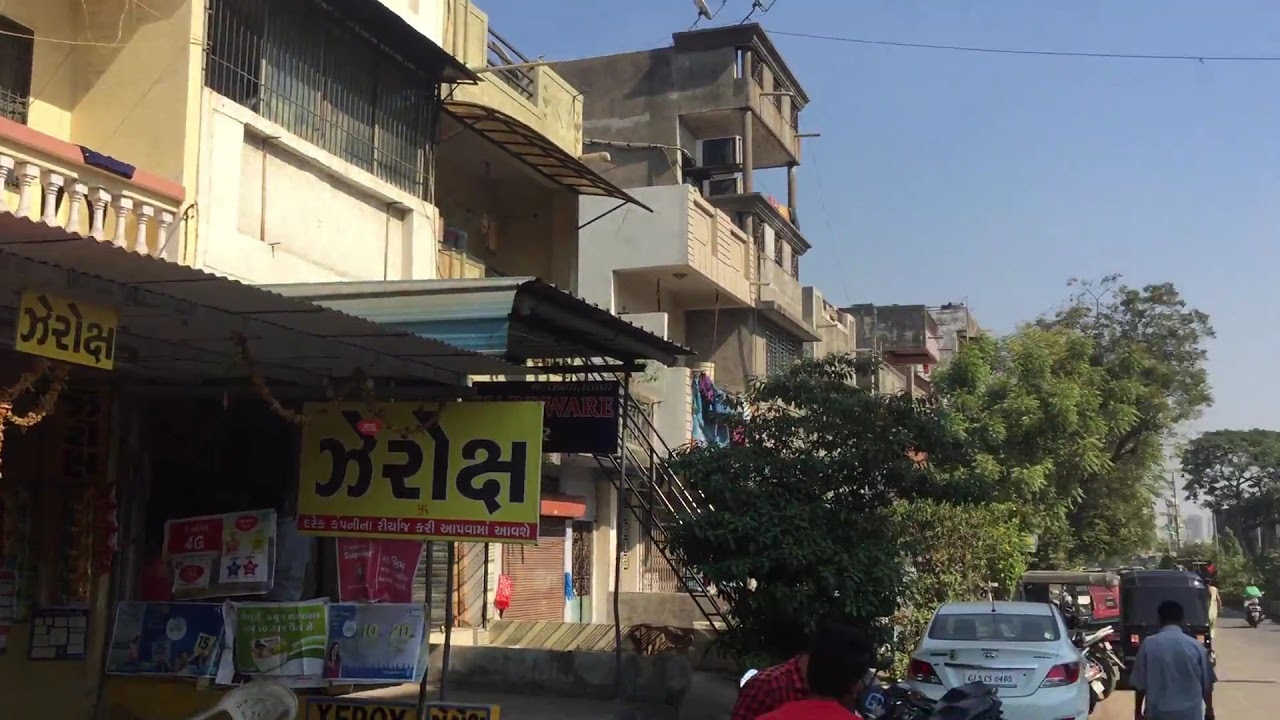The photograph captures a busy street scene in a vibrant Turkish city on a clear, cloudless day. The blue sky serves as a backdrop to a colorful and detailed urban environment. On the left-hand side, a series of multi-story buildings displays a mix of shops on the ground floors and residential apartments above, with porches featuring white columned railings and some contrasted by corrugated metal awnings. Signs and banners hang throughout, adorned with text in Turkish.

Tall, lush trees with green leaves line the space between the buildings and the street on the right. The street itself is bustling, with a variety of vehicles parked along it, including a blue car, a red car, a white car, mopeds, and what appear to be bicycle taxis with vinyl-covered roofs. Among the parked vehicles is a motorcycle situated in front of a white car. 

Visible in the lower right portion of the image is a person in a blue shirt with dark hair walking away, presumedly on the street beside a line of cars and a truck. Another individual, wearing a green shirt, appears to be riding a moped further down the right side. In the background, the tallest structure on the left side of the image appears to be a multi-story gray building with bare concrete walls.

Overall, the scene is filled with rich colors, including yellows, reds, blues, and greens, adding to the vivid and lively atmosphere of this Turkish street.